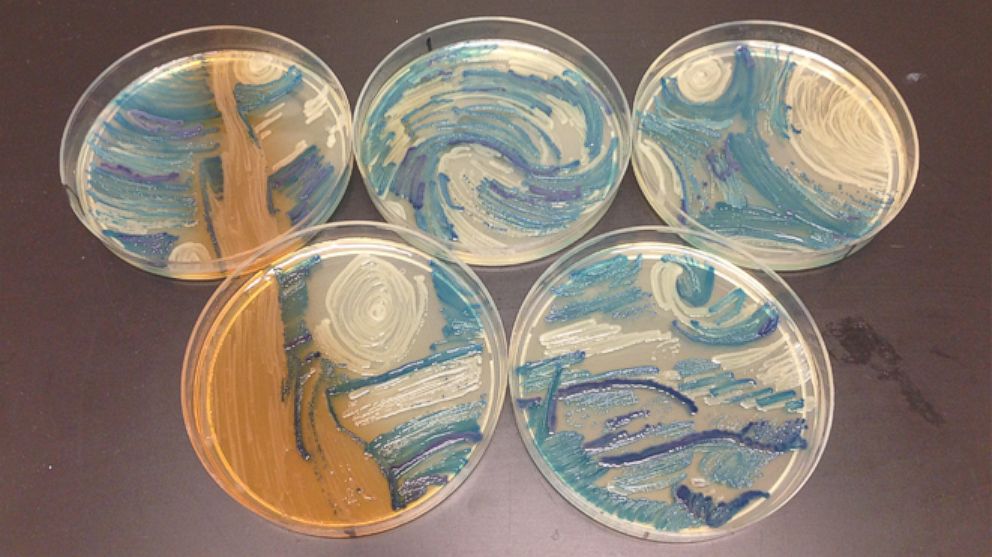This image features five small, circular glass dishes, arranged in a pattern reminiscent of the Olympic rings—with three dishes at the top and two below, each one touching the others. Set against a dark mahogany-colored background that resembles the surface of a table, the scene is illuminated by light shining on parts of the surface, giving it a dramatic contrast. 

The dishes, which could be mistaken for Petri dishes or small art receptacles, contain intricate abstract artworks. Upon closer inspection, these pieces appear to be painted, using swirls of various hues including dark blues, aquamarine, white, and hints of purple. Two of the dishes also incorporate brown, suggesting the form of a tree that spans from one dish to another, while hints of orange add a dynamic element to the pieces on the left.

The compositions within the dishes evoke a sense of nature and celestial imagery, resembling scenes from a starry night or abstract interpretations of mountain landscapes. The overall artistic arrangement, free of text or people, draws viewers into a close-up exploration of each dish, highlighting their colorful and swirling designs.